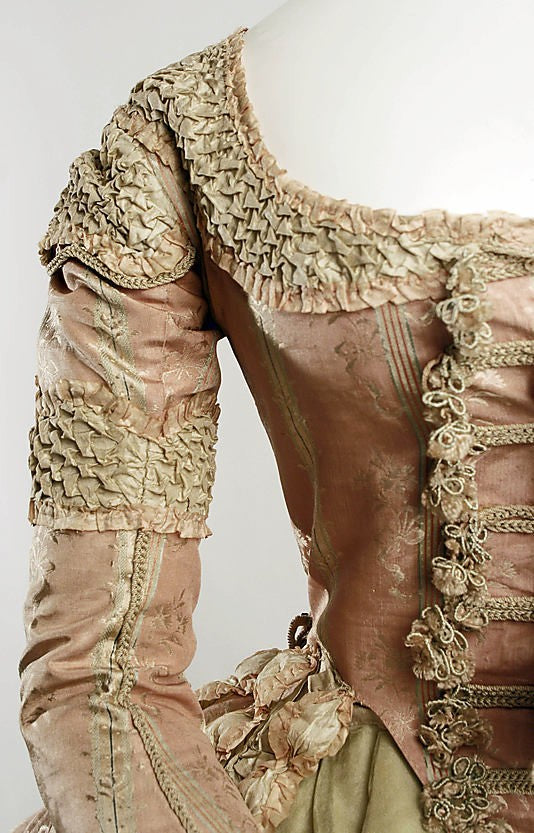This image showcases the right half of a vintage, ornate gown from what seems like the colonial or even earlier times, possibly dating back to the 1700s. The gown is displayed on a plain white plastic mannequin and features a tight bodice that transitions into a flared skirt with long sleeves. The gown, primarily in a faded pink silk, is richly adorned with gold embroidery and elaborately sewn gold ruffles, which are closely attached to the fabric, creating a textured pattern. These ruffles are accented by a rope-like gold trim that borders areas such as the bodice, sleeves, and neckline. The neckline and mid-forearm sections are decorated with overlapping, leaf-like fabric pieces. Despite its age and worn appearance, with colors fading into hues of light brown and hints of green at the bottom, the gown's intricate design and elegant adornments highlight the craftsmanship of the era.